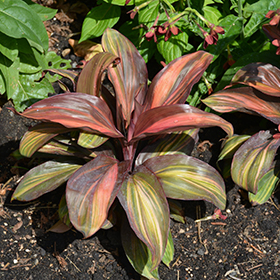This captivating outdoor photograph, bathed in sunlight from the right, showcases a lush, variegated flowering plant emerging from a textured ground of soil, mulch, and pebbles. The soil, which appears moist and contains small sticks, debris, and white pebbles, forms a rich brown canvas for the plant. The flowering plant itself is a mesmerizing tapestry of colors, with leaves striped in green, yellow, pink, brown, beige, red, and a hint of orange. The upper leaves transition into a striking maroon mix. In the background, vibrant green foliage provides contrast, interspersed with clusters of red berries and small red and purple flowers. The lighting highlights the intricate details and vivid hues of the plant, making it a clear and beautiful image despite its non-professional origins. The entire scene, devoid of any animals or text, focuses solely on the natural beauty and vibrant colors of the plant illuminated by the sun.